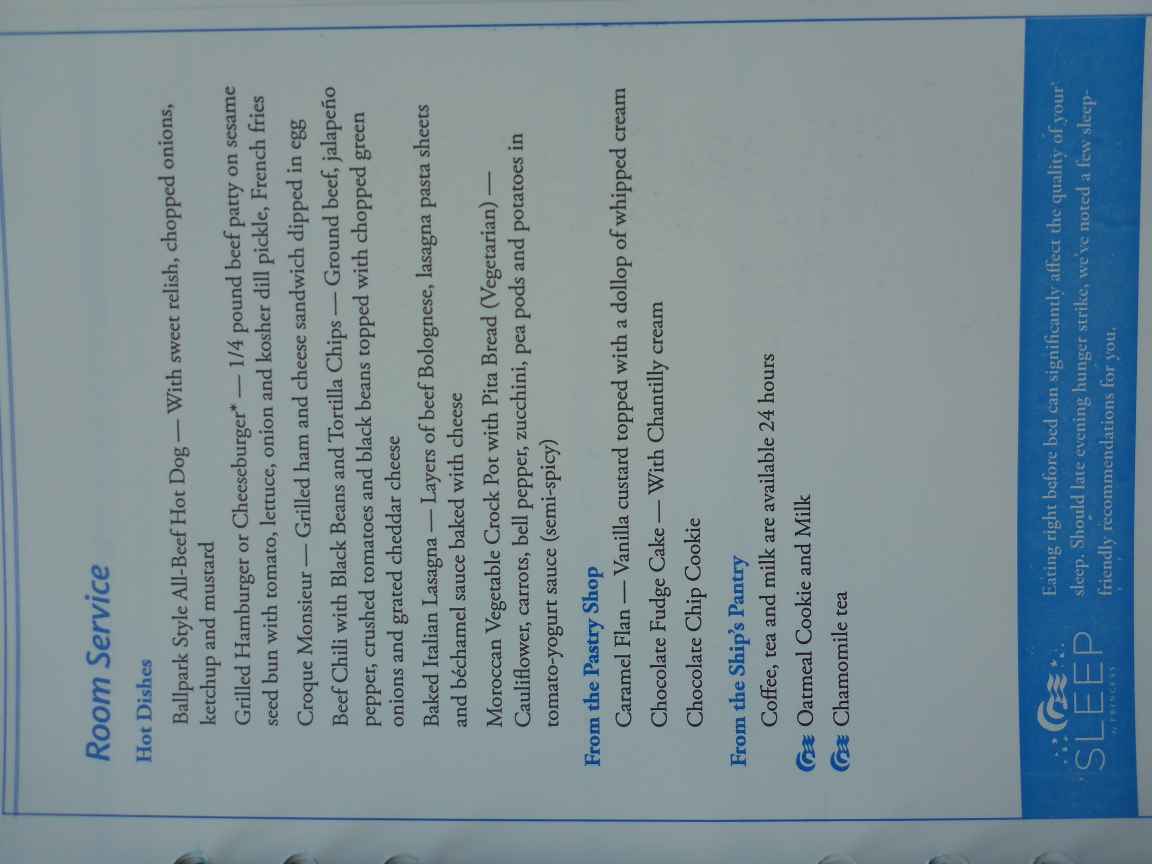The image displays a close-up of a room service menu, designed with black and blue text on white paper. At the top, the menu features the words "Room Service" prominently in blue. Following this, the subheading "Hot Dishes" introduces a list of savory options. 

The first item is a ballpark-style all-beef hot dog adorned with sweet relish, chopped onions, ketchup, and mustard. Next, the menu offers a grilled hamburger or cheeseburger made with a quarter-pound beef patty on a sesame seed bun, garnished with tomato, lettuce, onions, and a kosher dill pickle, accompanied by French fries.

Other delectable options include the Croque Monsieur, a grilled ham and cheese sandwich dipped in egg, and beef chili served with black beans and tortilla chips, enriched with ground beef, jalapeño peppers, crushed tomatoes, and black beans, all topped with chopped green onions and grated cheddar cheese.

The menu continues with additional items and culminates in a section highlighted in blue text titled "Pastry Shop," which includes a variety of desserts.